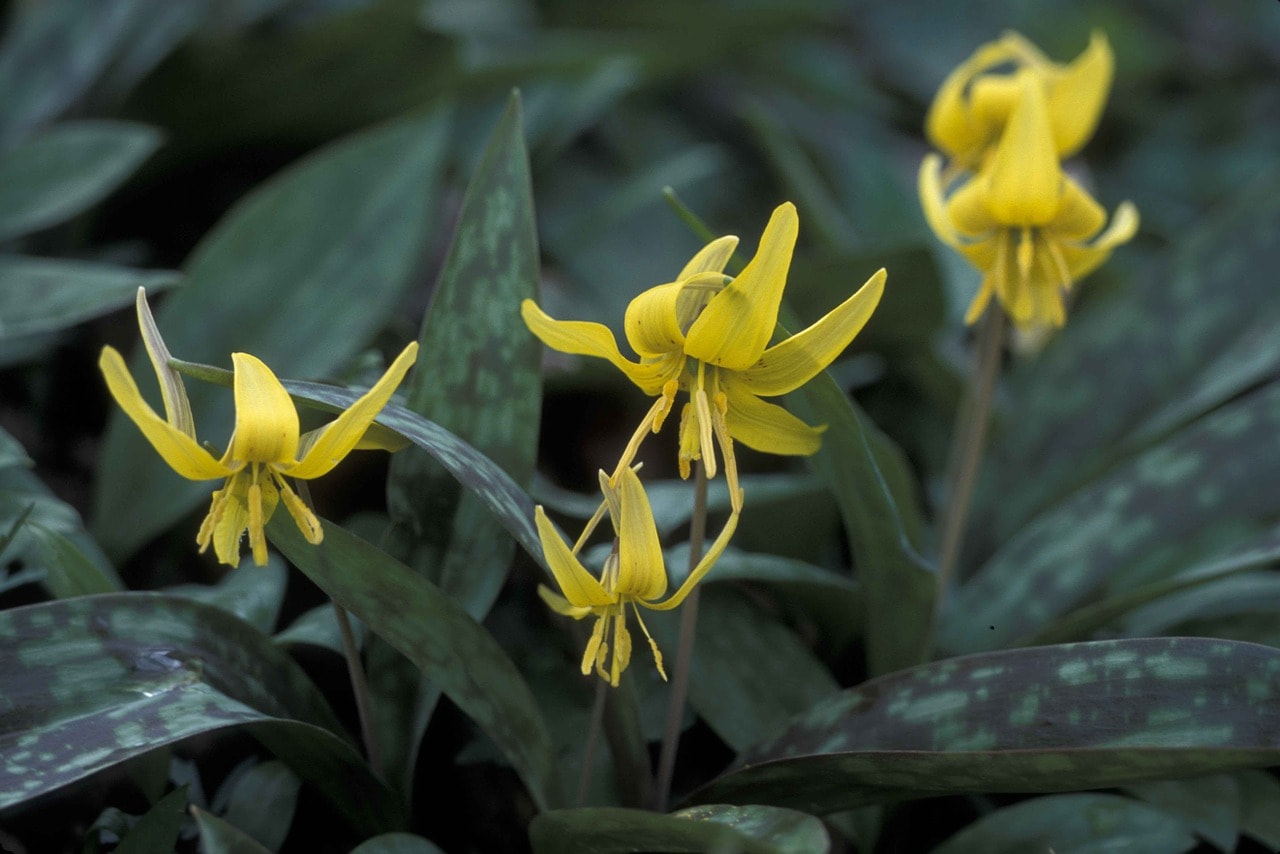This photograph, taken outdoors during the day, captures a close-up of four identical yellow flowers. Each flower droops downward, likely due to the weight of its curled-back petals and long filament, both of which are tinted yellow. They are supported by light brown stems that extend from a larger plant, which features thick, grass-like leaves streaked with gray and black spots. Surrounding these blooms are numerous leaves, some casting deep shadows, particularly from the left side and center behind the flowers. Due to the focus on the foreground, the background plants remain blurred, but it appears they are from the same plant, coexisting in a bed of greenery with faded hues.